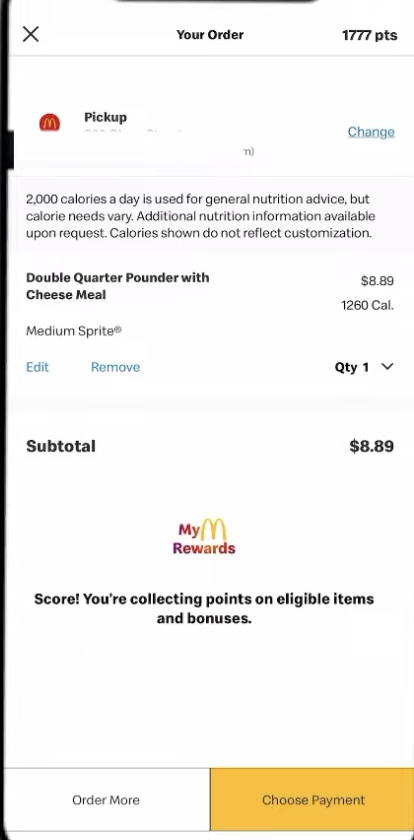A screen capture of a smartphone displaying the McDonald's MyReward app is featured in the image. At the top, the app indicates the user's current order and reveals they have accrued 1,777 points. Adjacent to this, there's an option for "Pick Up," accompanied by the iconic McDonald's logo. Users have the flexibility to change the pick-up location by clicking the “change” link. Nutritional information is visibly noted, advising that a daily intake of 2,000 calories is standard, but individual needs may differ. Customization may affect calorie counts. The user has ordered a Double Quarter Pounder with Cheese Meal totaling 1,260 calories, priced at $8.89. The subtotal is reaffirmed at $8.89. Below, under the “MyRewards” section marked with the McDonald's emblem, the app highlights the score, indicating points accumulation on eligible items and bonuses. Two prominent buttons offer options to "Order More" or "Choose Payment."